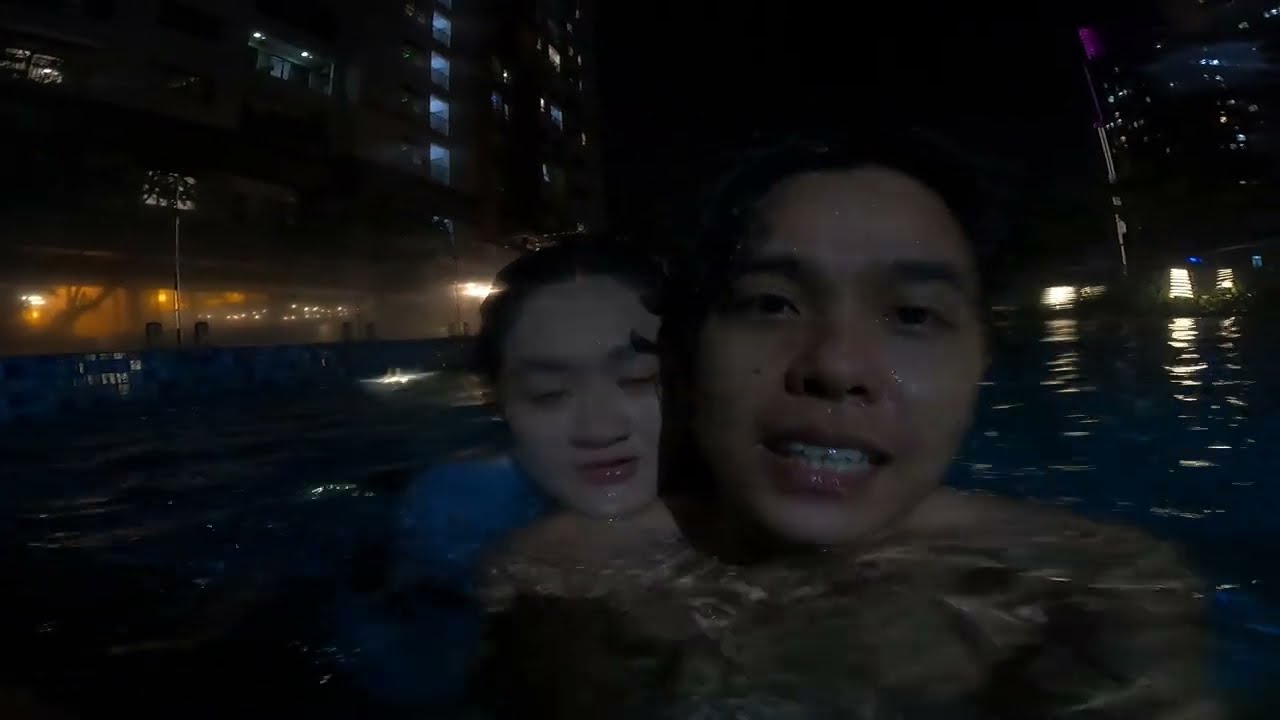This is an exterior nighttime color photograph capturing a close-up of two young, Asian individuals in a large, reflective pool, illuminated by surrounding city lights. The man, positioned closer to the camera with his face partially lit, is half-smiling with his mouth open, revealing both rows of teeth. He has dark hair that blends into the black night sky and no shirt on, visible beneath the water. The woman, resting her chin on his right shoulder, has long, dark hair, closed eyes, and slightly parted pink lips, and appears to be wearing a blue top. Behind them, the photo reveals the dimly lit expanse of the pool and the silhouettes of tall buildings, their lights casting a soft, yellowish glow on the rippling water's surface. The black background accentuates the nighttime ambiance, making their figures appear as shadowy silhouettes against the dim illumination of the urban landscape.